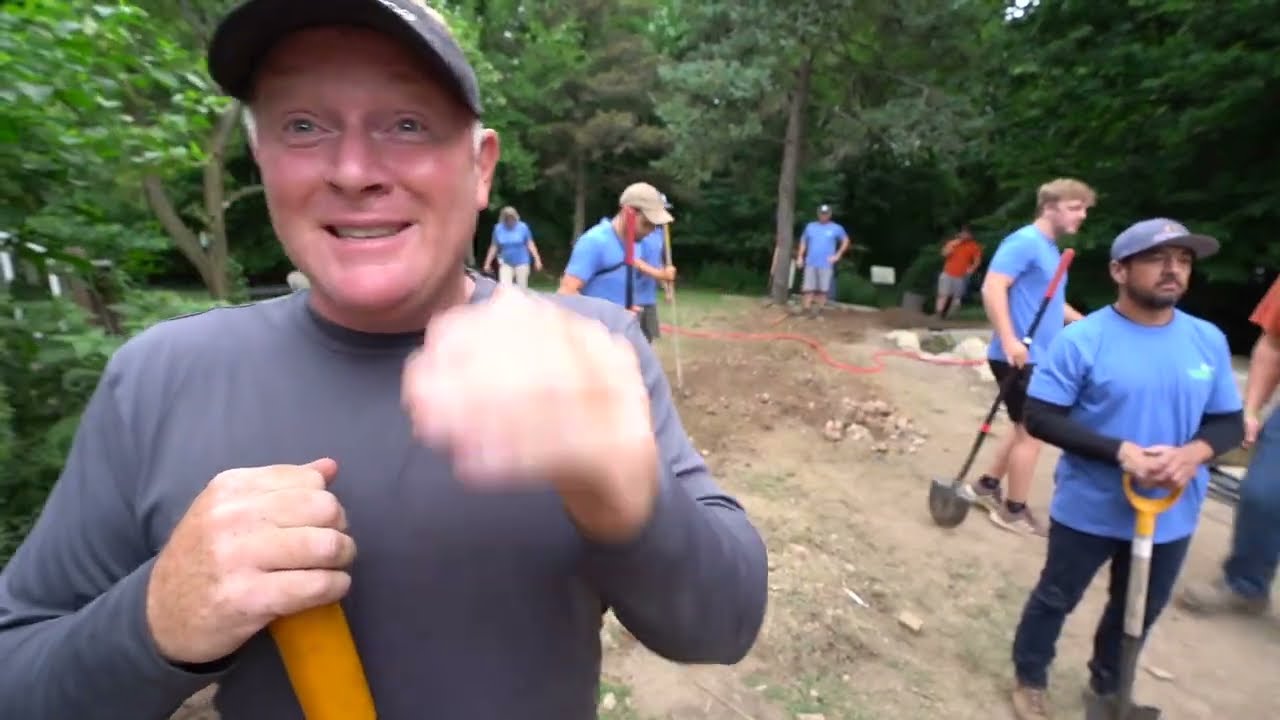Amidst a serene outdoor setting characterized by a dirt clearing surrounded by lush, green trees, a diverse group of individuals is engaged in excavation or cleanup work. Dominating the left foreground of the picture, a cheerful, white-haired man with a baseball cap and a grayish-blue long-sleeved shirt, smiles warmly while his left hand—blurred from motion—is raised beside his face. His right hand firmly clutches a yellow-handled shovel. Scattered around him are men and women of various ages, most of whom are clad in blue t-shirts, with a few in red and orange shirts visible. In particular, a man slightly to the right of the center wears a blue short-sleeve shirt over a darker undergarment, a blue cap, and jeans, while holding a shovel. Another person behind him in a tan cap and blue shirt, also wielding a shovel, is engaged in the same activity. A red cord zigzags across the image, indicating the organized nature of their project. The scene encapsulates a collaborative spirit with participants engrossed in their shared work, enhancing the natural environment around them.